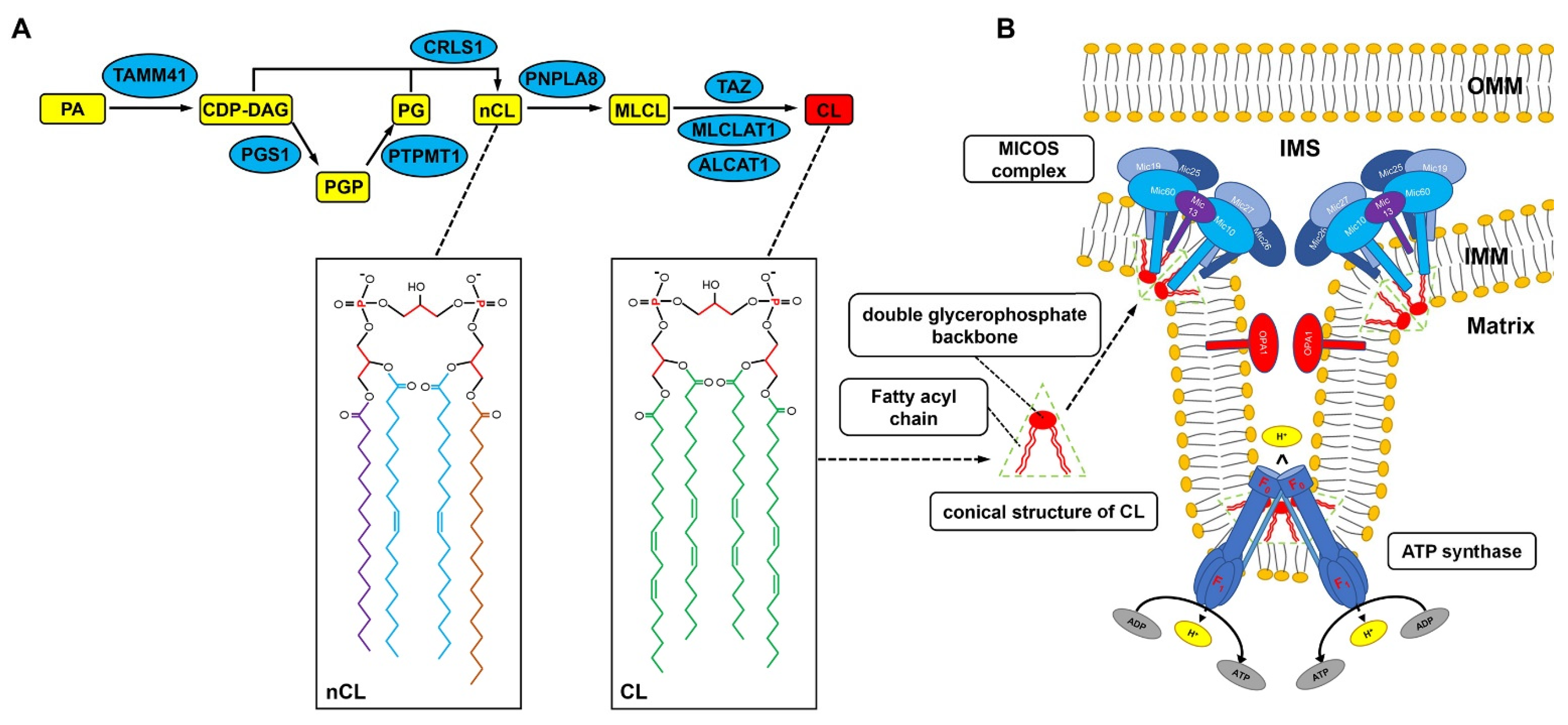The image is a detailed diagram likely from a science textbook, possibly in the fields of biology or chemistry. The layout is divided into two main sections, labeled A on the left and B on the right. In section A, a flowchart displays a process using various shapes in primary colors: yellow rectangles and blue ovals. The flowchart begins with the abbreviation "PA" and follows with arrows to "CDP-DHE," "PGP," "PG," "NCL," "MLCL," and ends at "CL." Adjacent to the flowchart are two squares, each containing the labels "NCL" and "CL," respectively.

Section B presents a schematic of cellular structures or processes, containing terms like "mycose complex," "double glycerophosphate backbone," "fatty acyl chain," "conical structure of CL," "ATP synthase," "matrix," "IMM," "IMS," and "OMM." The diagram is visually engaging, made with simple primary colors, and features significant scientific annotation, indicating its educational use in explaining complex biological or chemical processes.